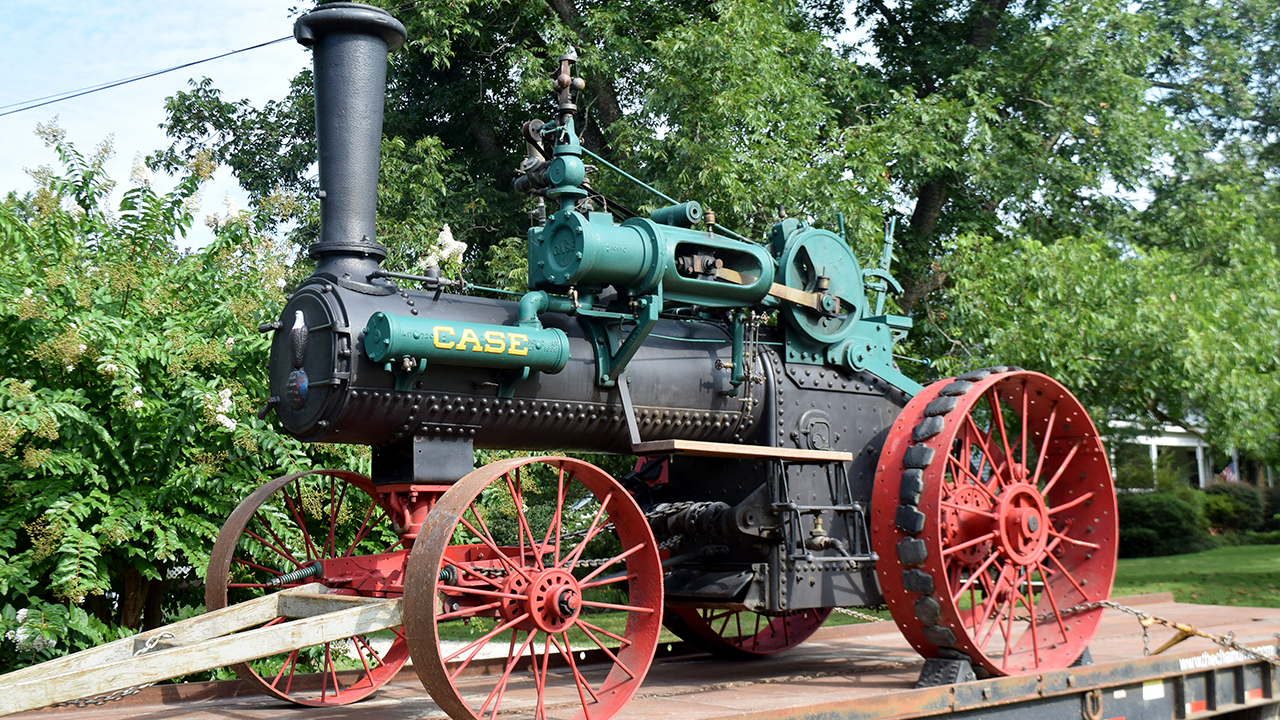This photograph captures a detailed and well-maintained old-fashioned steam engine from the 1800s or 1700s, mounted securely on a flatbed truck. The centerpiece of the image is the steam engine itself, which features a black body with green piping and machinery. Prominently displayed on a green cylinder, the word "CASE" is emblazoned in yellow, vintage-style lettering. The engine has four sizeable, iron-spoked red wheels, with the front wheels resting on a small wooden frame made of 2x4s to keep it stable during transport. The background reveals a rural setting with lush greenery, including large oak trees, bushes, some grass, and a glimpse of a white house or building. Overhead, an electric line stretches across a light blue sky dotted with occasional white clouds. The steam engine is fitted with a black smokestack and various riveted components, evocative of its historical significance as one of the first steam-powered engines. The entire scene is illuminated by clear, bright daylight, adding to the sense of nostalgia and preservation.